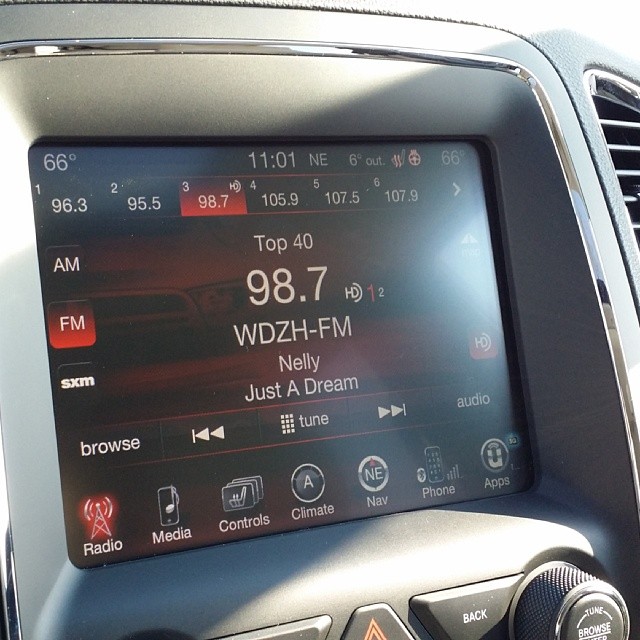This detailed image showcases the infotainment system of a car's dashboard. Central is a large, probably touch-sensitive, digital screen framed by the plastic outer area of the dashboard. In the top left corner of the screen, it displays the temperature as 66 degrees, and just below that, the time reads 11:01. The screen also highlights the car's bearing of northeast, and 6 degrees.

The primary focus is on the audio system, specifically tuned to the radio station 98.7 WDZH-FM, which is prominently displayed with a red background, indicating it's the active station. It is currently playing "Just a Dream" by Nelly. Other preset stations, numbered 1 through 6, include 96.3 and 95.5. The controls offer diverse functionalities, featuring AM and FM buttons on the screen, as well as physical analog knobs below sound-tuning labeled "tune/browse."

At the screen's bottom, several touch-sensitive icons are visible, dedicated to radio, media controls, climate, navigation, phone, and apps. The screen's interface is designed with a mix of red and black accents, adding to the modern and sleek aesthetic. Also noticeable is a vent located to the upper right side of the screen, likely the passenger-side vent depending on the car's orientation.

Other notable physical buttons include a back button and an emergency light button situated below the screen, ensuring essential vehicle controls are easily accessible. Overall, the detailed image captures the elaborate and user-friendly design of the car's infotainment system, providing both functionality and a refined interface.